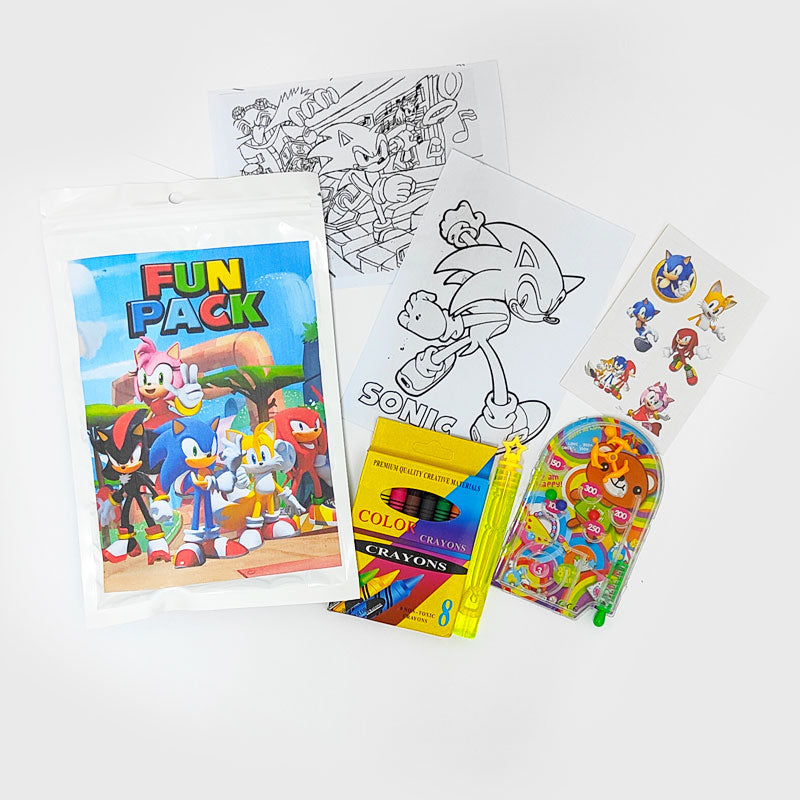This image shows a Sonic the Hedgehog Fun Pack laid out on a white background, perfect for young fans of the video game series. The Fun Pack itself is a white or off-white Ziploc bag with a hole at the top for hanging. On the front of the bag, there is a colorful, rectangular illustration featuring Sonic and his friends with the words "Fun Pack" written in bright, multicolored letters—red, green, yellow, blue, and light blue.

To the right of the Fun Pack, the contents are carefully arranged. There are two black-outline coloring pages typical of a coloring book. One page features Sonic running to the right with Dr. Robotnik in pursuit, evoking a sense of dynamic action, even showing Sonic running over piano keys with musical notes in the upper right corner. The second page showcases Sonic walking away from the viewer, labeled "Sonic" underneath, with Sonic glancing back over his shoulder.

In addition to the coloring pages, there is an 8-pack box of crayons, standing ready to bring the drawings to life with color. A small yellow bubble wand with a star-shaped top sits nearby, promising hours of bubbly delight. Also included is a small, plastic-covered silver bead game with teddy bears in the background and red circles with point values, adding a playful touch. Finally, there is a sheet of six pre-colored stickers featuring various Sonic characters, providing immediate vibrant excitement to young Sonic enthusiasts.